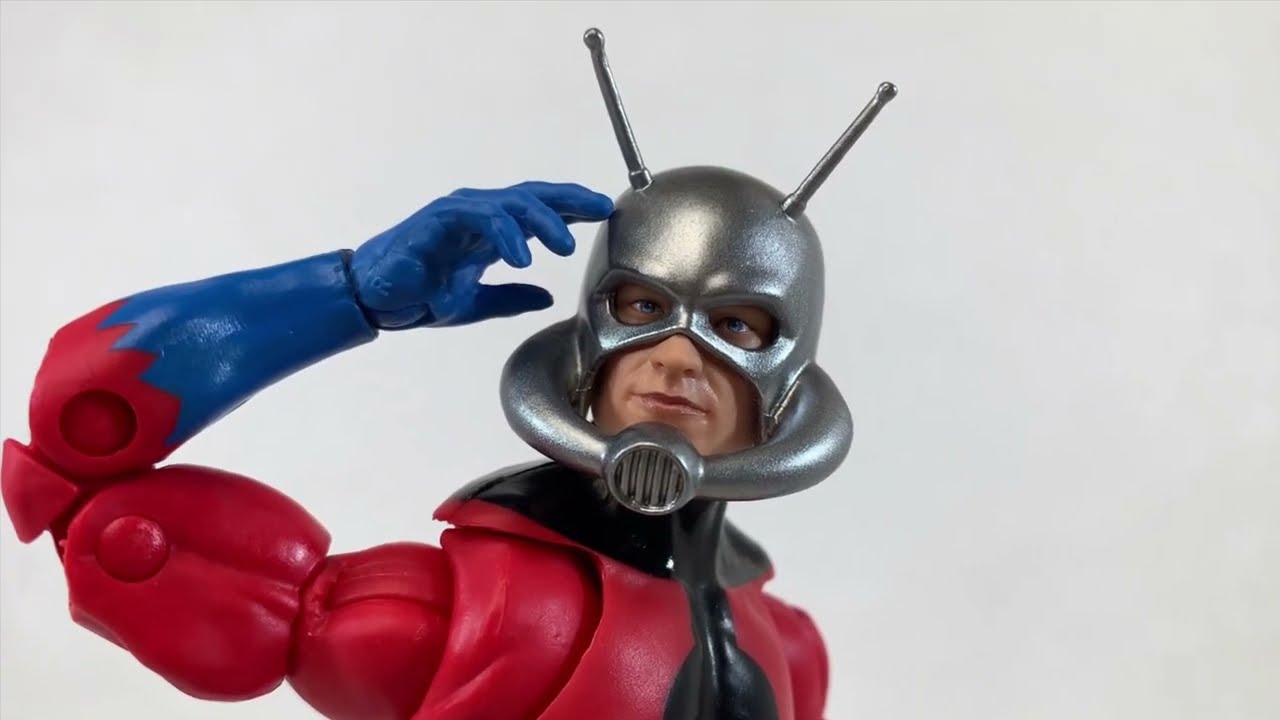This detailed caption integrates elements from all three voice descriptions:

The image features a highly detailed action figure, seemingly from a popular TV series or movie, captured against a plain white background. The figure portrays a muscular man adorned in a distinctive red and black outfit, with a red torso having a black collar and black front section. One unique attribute is his right arm, which transitions from red to blue just below the elbow and continues to his fingers. The intricate elbow joint is visibly designed with multiple circular hinges and a wedge part, indicating its poseability.

The figure's head is equipped with a prominent silver or grey helmet, equipped with three antennas—two protruding sideways from the helmet and one on the top. Notably, the helmet also includes a microphone-like extension in front of his mouth. Facial details are partially visible through the gaps in the mask, exposing the mouth and nose while the eyes are covered. The figure's pose has his arm bent upwards towards his head, almost as though he is giving a salute or pointing at his helmet. The high degree of detail and specific features, such as the unique color scheme and articulations, suggest this could be a classic or vintage character, possibly reminiscent of an old comic book or sci-fi series.